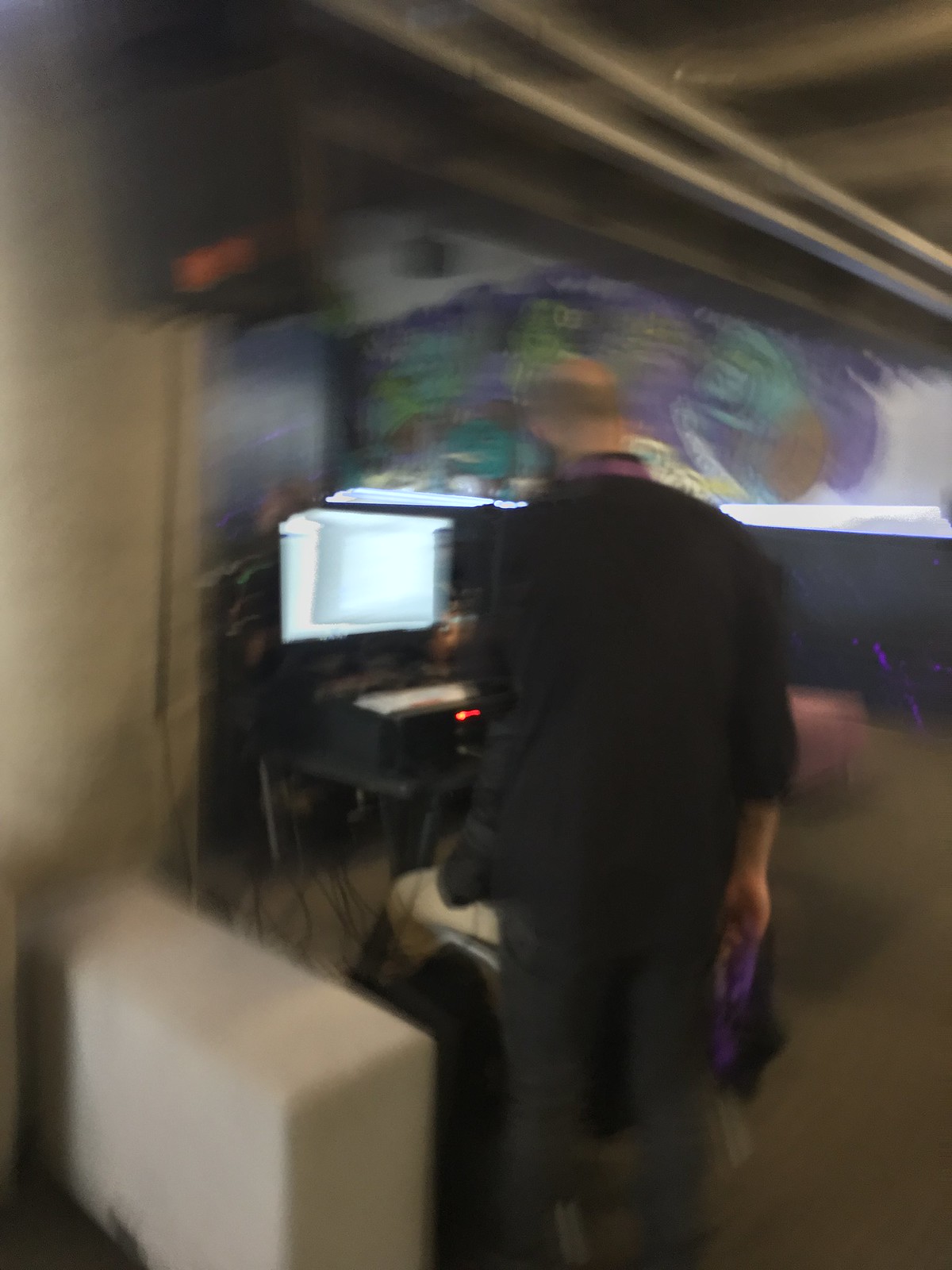In this slightly blurred image, we observe a man with a shiny bald head and some hair around the sides, dressed entirely in black, including a collared shirt and black pants. He is standing in front of a computer monitor on a wall-mounted desk, within a spacious room that resembles an office. He holds a black and purple object in his right hand, while his left arm is obscured, possibly supporting a shoulder bag that blends into his attire. The desk, attached to a cream-colored wall, features a multitude of wires descending behind it. Just beside the desk, there is a small white protrusion from the wall, likely a piece of furniture or a low wall divider. The man, standing as if speaking to someone possibly seated at the desk, blends into the surrounding backdrop that includes overhead pipes, likely for water, and rows of fluorescent lights running at an angle from the top center towards the right. The ceiling, punctuated with these lights, and the medium brown floor complete the setting. In the distance, an indistinct mural or image exhibits a medley of colors including purple, green, teal, brown, and white, further adding to the complexity of the scene.